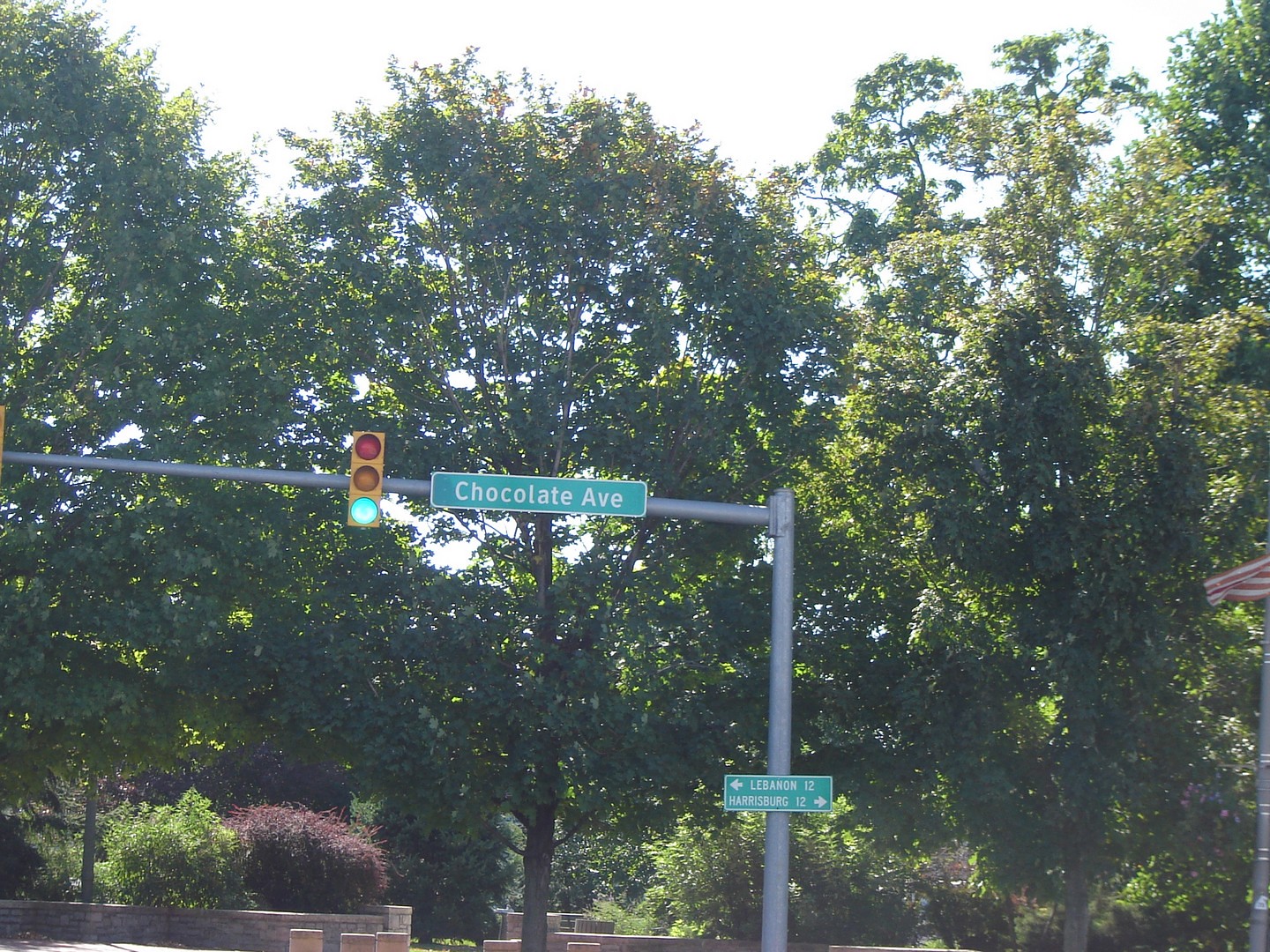In this outdoor image, the setting takes place in a scenic park, characterized by lush green trees forming a dense backdrop. A prominent feature in the foreground is a traffic light mounted on a robust metal post. Extending horizontally from the main post is an arm that supports both the traffic light and two street signs. The traffic light is clearly illuminated with a vibrant green signal. Adjacent to the traffic light, a green sign boldly displays the street name "Chocolate Avenue." Positioned midway down the post, a directional sign provides further guidance: it indicates "Lebanon 12" with an arrow pointing to the left and "Harrisburg 12" with an arrow pointing to the right. The well-maintained appearance of both the signage and the surrounding park highlights the blend of natural beauty and orderly infrastructure in this area.